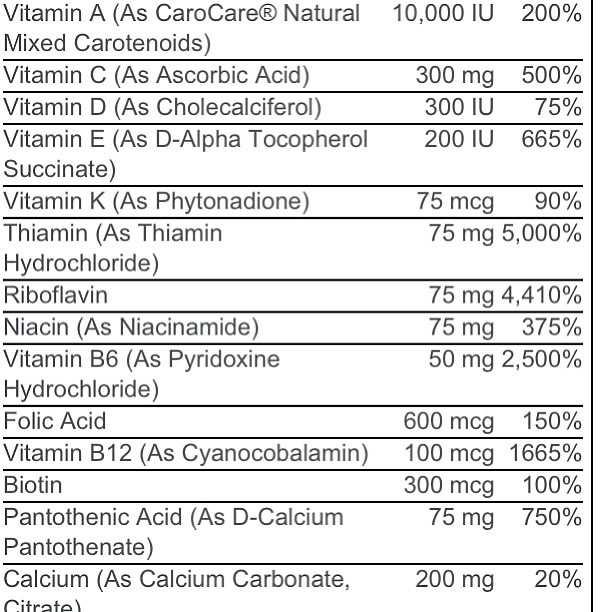The image features a square-shaped, white background dominated by a list of nutritional facts written in English with black text. A vertical thin black bar runs along the far right side of the image. The nutritional information is organized meticulously, with each nutrient's details separated by thin horizontal lines. At the top of the list, it states:

- Vitamin A (as carotenoids): 10,000 IU (200%)
- Vitamin C (as ascorbic acid): 300 mg (500%)
- Vitamin D (as cholecalciferol): 300 IU (75%)
- Vitamin E (as D-alpha tocopherol): 200 IU (665%)
- Vitamin K (as phytoaddenone): 75 mcg (90%)
- Thiamin (as thiamine hydrochloride): 75 mg (5,000%)

The list continues in a similar format, specifying each nutrient along with its respective amount and daily percentage value. There are approximately 20 nutrients detailed in the list, each with specific information about its composition and nutritional value.